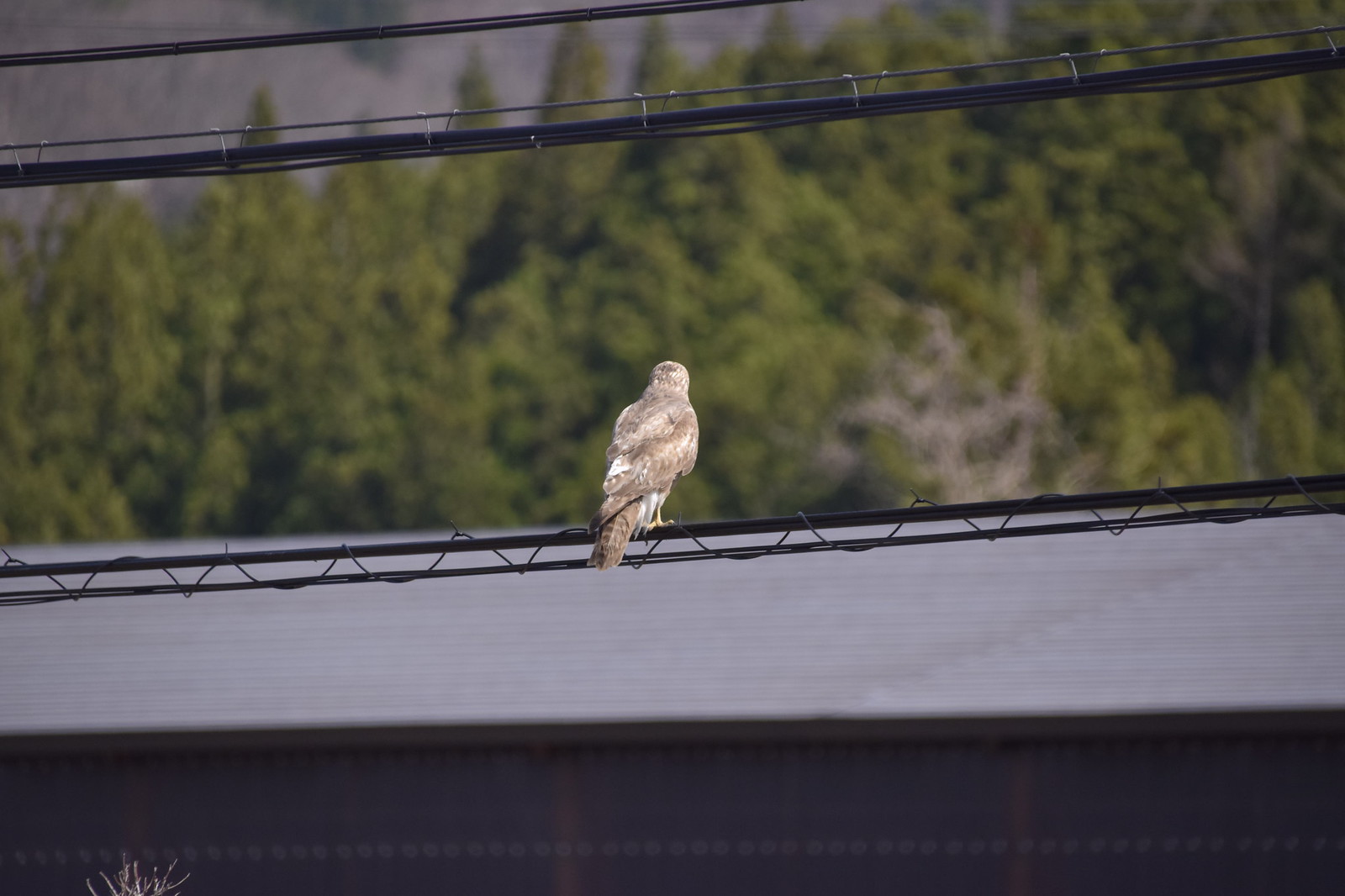The image captures a small brown bird with some white markings, perched on a pair of power lines in a sunny, outdoor setting. The bird is facing away from the camera, so only its back and long feathers are visible. Its yellow feet grip the power lines, which glisten with the sunlight. The background features green trees and a grey building, partially obscured by the shallow depth of field, while distant mountains add depth to the scene. An additional power line is faintly seen parallel to the ones the bird is perched upon. The high-quality photograph emphasizes the bird and power lines, leaving the environment slightly blurred but still discernible.